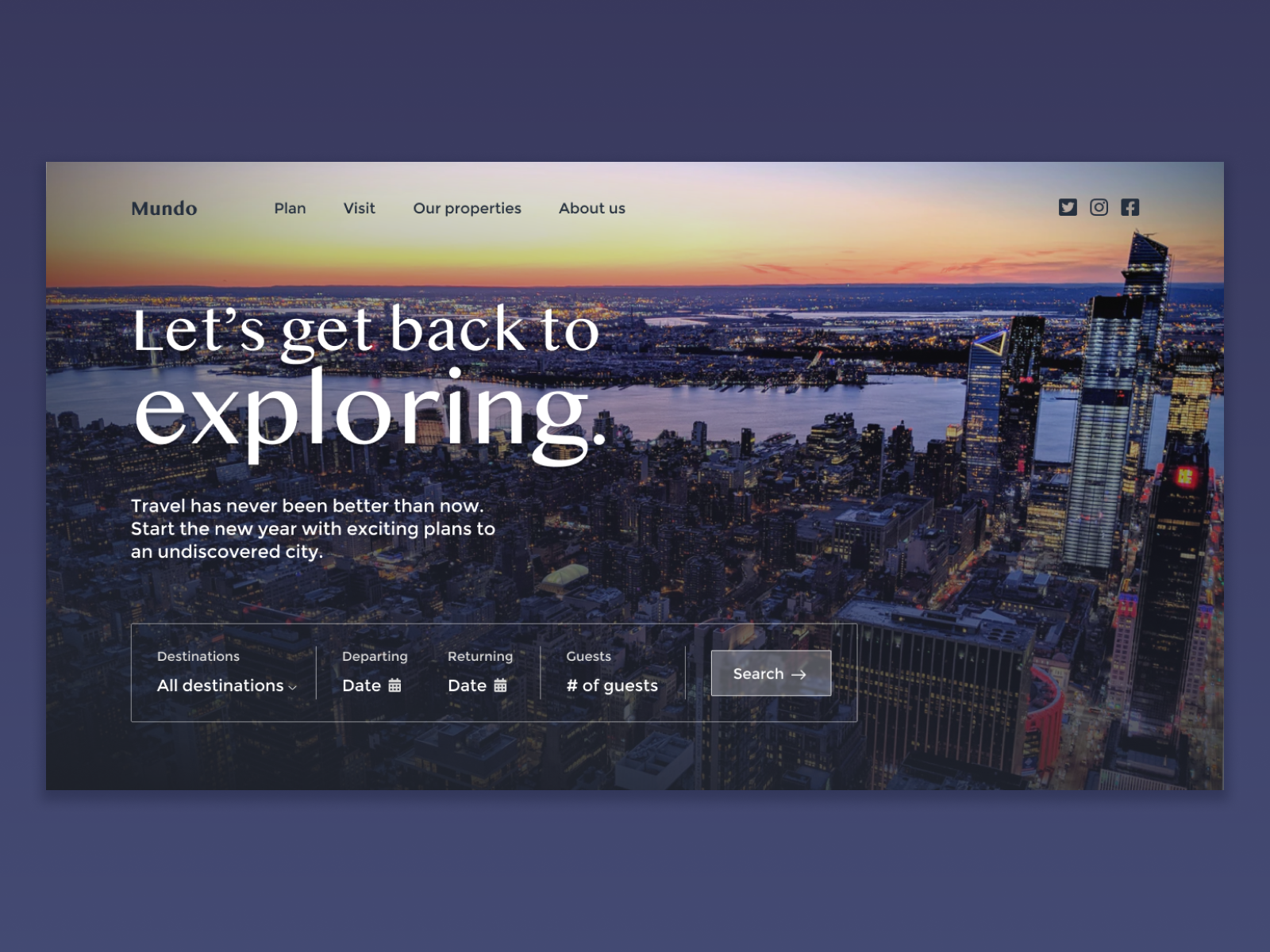This landscape-oriented image showcases a travel website with a gradient blue background, transitioning from a darker shade at the top to a lighter hue towards the bottom. Dominating the center is a large box featuring a stunning cityscape at sunset. The sky is awash with vibrant shades of orange, yellow, and blue, casting a beautiful glow over the bustling metropolis, teeming with lights and silhouetted tall buildings against serene waterways.

In the top left corner, the bolded black word "Mundo" stands prominent. Adjacent to it are navigation options including "Plan," "Visit," "Our Properties," and "About Us," with social media icons for Twitter, Instagram, and Facebook aligned to the right. 

On the middle left of the image, white text beckons with an inspirational message: "Let's get back to exploring. Travel has never been better than now. Start the new year with exciting plans to an undiscovered city." 

Below this message is a functional white text box segmented into smaller interactive fields. These include a dropdown menu labeled "All Destinations" with a caret, fields for selecting "Departing" and "Returning" dates, and a section for specifying the number of guests. All of this is accompanied by a transparent gray search button outlined in white, inviting users to commence their travel planning. Every detail suggests an invitation to explore and tour new exciting areas.